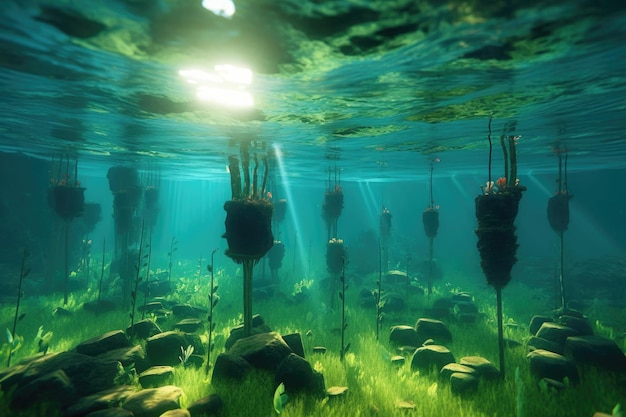This underwater scene showcases a rich, detailed aquatic ecosystem. At the bottom, a mix of smaller rocks and tiny green plants create a textured bed. Tall, thick, trunk-like plants dominate the middle of the image, shooting up from the bottom and winding through the water towards the surface, where they disperse into a nest-like formation holding additional flora. The water is a vibrant blue, and sunlight pierces the surface from the left middle area, casting a warm glow through the green aqua-colored moss floating near the waterline. Shadows and light interplay as the bright glare on the left contrasts with the darker tones towards the top left of the image, highlighting the dynamic, layered nature of this underwater habitat.